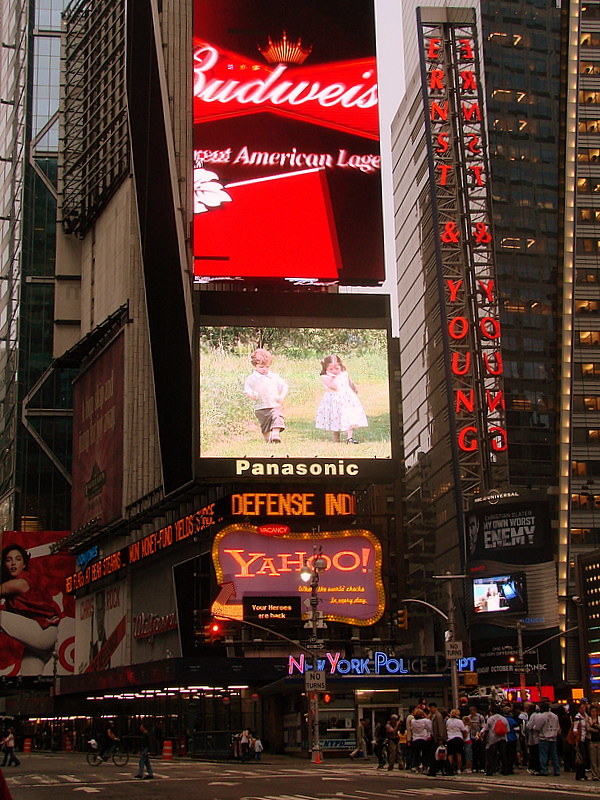This captivating photograph showcases the vibrant heart of Times Square, New York City, bustling with illuminated billboards and neon lights. Dominating the scene at the top is a striking Budweiser billboard in bold red, flaunting the iconic Budweiser logo with the inscription "American Lager." Directly below it, a Panasonic jumbotron displays a serene video of two toddlers, a boy on the left and a girl on the right, strolling through a grassy field. Beneath this screen is a prominent Yahoo advertisement with a purple background and a shimmering gold border. Further down, the New York Police Department is signified by an illuminated sign, with "New York" in vivid neon lights, red for the 'N' and 'Y,' and the other letters in blue. To the right of this sign, a crowd of people is gathered, adding to the bustling atmosphere. High-rise buildings frame this lively cityscape, including the recognizable Ernst and Young building, its name emblazoned on scaffolding. This quintessential Times Square snapshot is a testament to the area’s dynamic energy and iconic advertising allure.